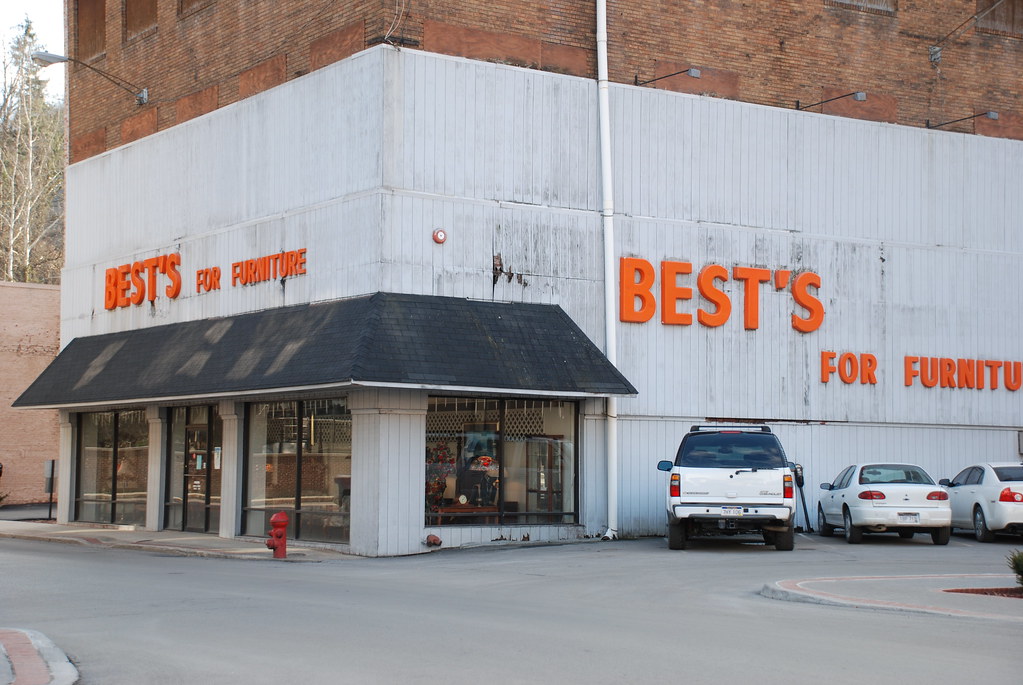The photograph captures the exterior of a store named "Best for Furniture," characterized by an orange sign with the store's name. The establishment is located on the ground floor of a dull gray building, possibly with apartments above, although the upper portions of the structure are not fully visible. The right-hand side of the image showcases a gray parking lot, where three white vehicles are parked, including a truck and two sedans. The truck has indistinguishable license plates with blue and yellow elements. In front of the store, there is a fire hydrant and four large, black-framed glass windows. A street light is fixed to the side of the building above the ground floor, attached to what appears to be a brick section of the structure.